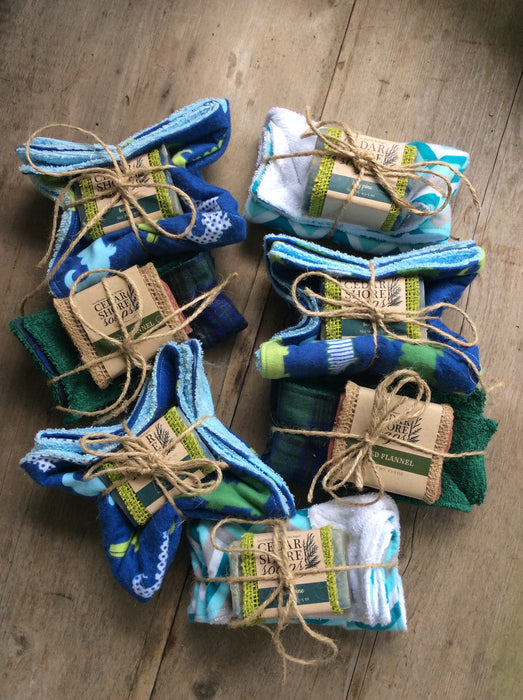The image shows an overhead view of a wooden floor adorned with seven neatly arranged packages, each comprising a bar of Cedar Shores Soap wrapped in variously colored towels. These towels, possibly hand towels or washrags, include colors such as blue, green, light blue, and white. Each bar of soap is wrapped in burlap with a beige label bearing the brown text "Cedar Shores Soaps" and a green box with unreadable text. The soap packages are secured with a light brown drawstring, likely jute, that elegantly ties them to their respective towels. The arrangement includes a variety of towel colors and patterns: blue and green, light blue, dark green bordered in blue, and even a smaller all-green towel. The bottom-most towel is unique with its white and light blue design. This visually cohesive display effectively blends rustic and colorful elements against the wooden backdrop.